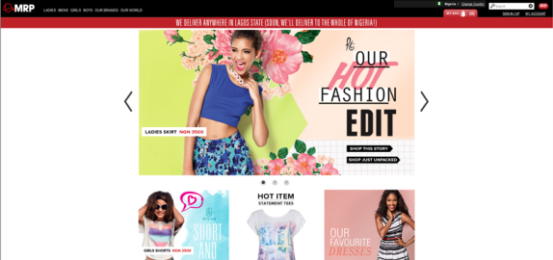The image depicts the homepage of MRP (Mr. Price), a fashion retail website identifiable by its red hat logo. Dominating the page is a bold banner proclaiming "We Deliver Anywhere," highlighting their delivery service across Nigeria. The banner also features promotional images, including a vibrant photograph of a light-skinned woman joyfully modeling colorful attire, representing 'Our Hot Fashion Edit.' Below the banner, several more images showcase a diverse range of fashionable clothing items available for purchase.

At the top of the page, a series of navigation buttons are visible, providing users with various browsing options, although the text of these buttons is too small to be legible in the image. Additionally, a search bar is prominently placed, enabling users to quickly find specific items. Despite the vibrant promotional images, the overall design of the site appears quite plain and straightforward.